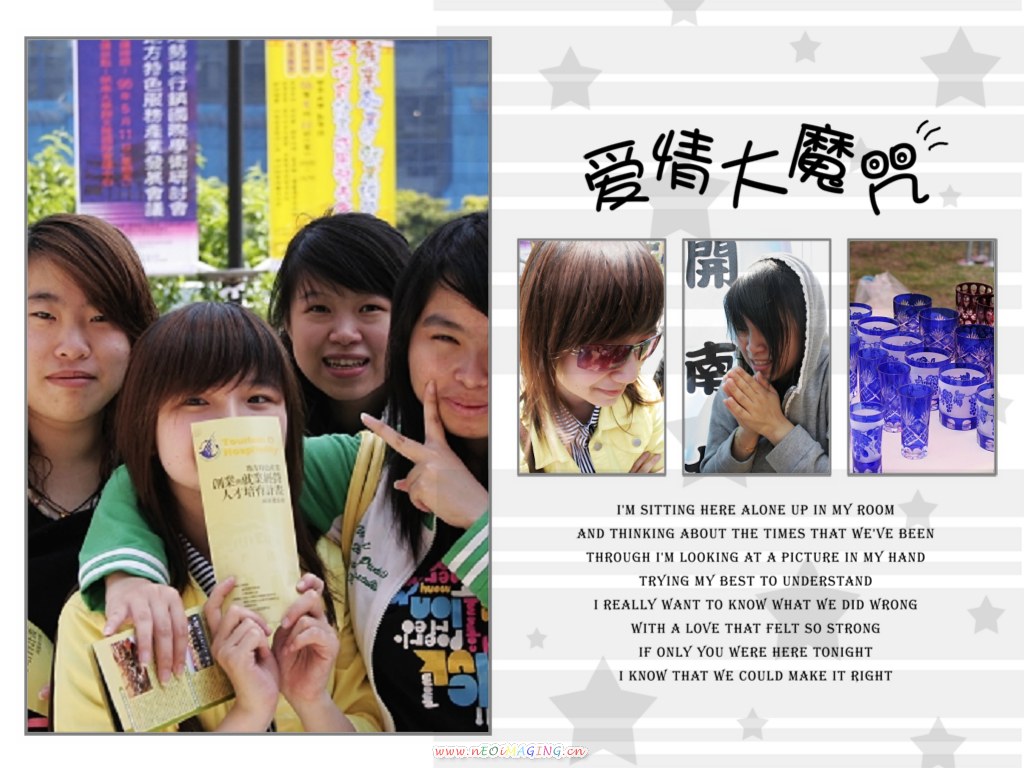The image is a composite of two photographs side by side. The left photograph depicts four women with dark hair and bangs, positioned against a backdrop featuring signs with Asian text in blue, yellow, and red. The woman on the far left is making a peace sign, while the woman in the center partially obscures her face with a yellow brochure. Behind them, a modern building and some trees can be seen. The right photograph is set against a gray background decorated with white stripes and stars. It features three smaller images: the first shows a woman wearing sunglasses, the second captures a woman in a gray hoodie with hands folded in a prayer-like position, and the third displays a group of blue cups. Below these images is a caption that reads, "I'm sitting here alone up in my room and thinking about the times that we've been through. I'm looking at a picture in my hand trying my best to understand. I really want to know what we did wrong with the love that felt so strong. If only you were here tonight I know that we could make it right."